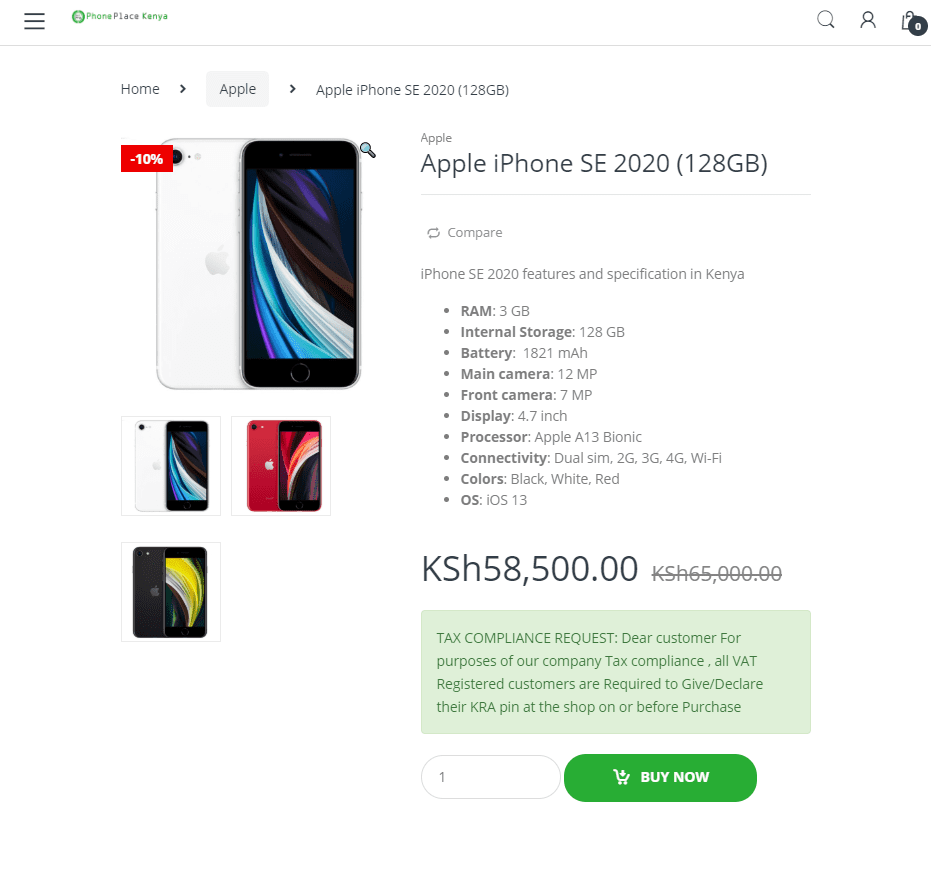This screenshot from the Phone Place Kenya website details the Apple iPhone SE 2020, 128GB model. At the top left corner, the website's name, "Phone Place Kenya," is displayed. On the top right, icons for search, login, and shopping bag are visible. Below, navigational elements list "Home," "Apple," "Apple iPhone SE 2020," and "128 gigabytes."

The image showcases both the front and back views of the white iPhone SE 2020. A "10% off" tag highlights the discounted price. The device's detailed features and specifications are listed: RAM of 3GB, internal storage of 128GB, a battery capacity of 1821 mAh, a 12 MP main camera, a 7 MP front camera, and a 4.7-inch display powered by the Apple A13 Bionic processor. Connectivity options include dual SIM, 2G, 3G, 4G, and Wi-Fi. The available color options are black, white, and red, and the operating system is iOS 13.

To the left, additional images display the phone in black and red colors. The current price is shown as KSH 58,500, marked down from KSH 65,000. A tax compliance notice at the bottom informs customers to declare their KRA PIN at the shop for VAT registration before purchase.

At the bottom, there is an option to "Buy Now."